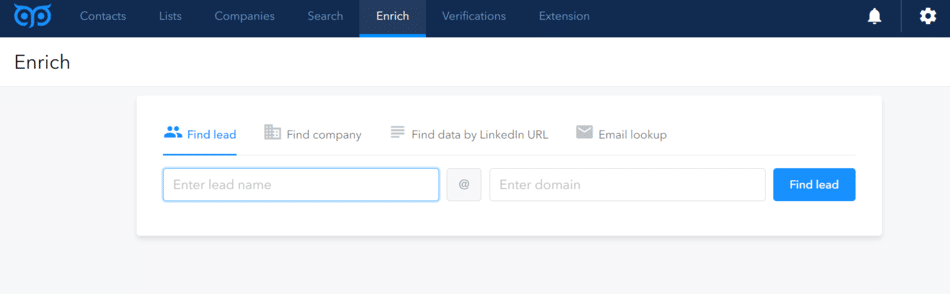This image depicts a simplistic web interface resembling a software application for lead enrichment. Dominating the top is a blue navigation bar, adorned in the upper left corner with a blue owl face icon, symbolizing the brand or platform. To the right of the owl icon, a series of clickable menu items are arranged: Contacts, Lists, Companies, Search, Enrich, Verifications, and Extension. The 'Enrich' option stands out with a white background and a blue underline, indicating it has been selected.

Beneath the owl logo and within the main white content area, the word "Enrich" is prominently displayed. The page layout features a central gray box framing a long, slim, horizontal white rectangle. Within this rectangle, a blue-underlined prompt reads "Find Lead." Directly beneath is another interactive element: a white box bordered in blue, prompting users to "Enter Lead Name." Adjacent to this, an icon of the at-symbol (@) is displayed to guide the input format. Following this, a gray rectangle instructs users to "Enter Domain." To finalize the search, a small blue rectangle labeled "Find Lead" is positioned to the right, serving as the actionable button for initiating the lead search process.